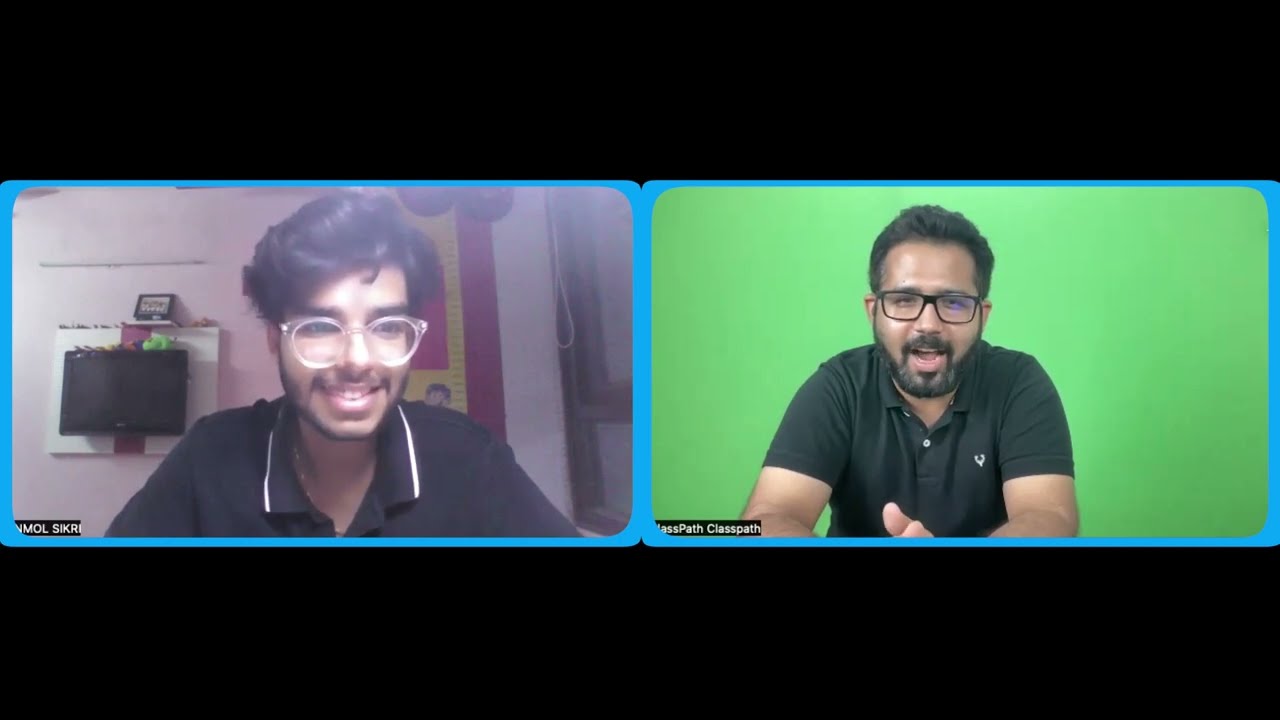This image appears to be a screenshot from a virtual meeting, likely conducted over platforms such as Zoom or Skype. The image features two men side by side at the center, each outlined in blue against a black background with splashes of colors including black, white, gray, pink, blue, green, red, and yellow. 

The man on the left has fluffy black hair and is wearing large, round, clear-framed glasses. He is dressed in a black collared shirt with white accents on the collar. He has a slight mustache and is smiling. His background is somewhat unclear, though it appears to be a room with items on the wall that are not clearly identifiable.

The man on the right dons dark-framed glasses and has black hair, tan skin, a beard, and a goatee. He is also dressed in a black shirt with a black collar, but without white accents. Behind him is a green screen. Unlike the man on the left who is smiling, the man on the right seems to be mid-sentence.

The overall impression is that both individuals are engaged in a virtual conference, with the precise text on the image being too tiny to read. Their composed and expressive demeanors suggest an active communication scenario, typical of virtual meetings.